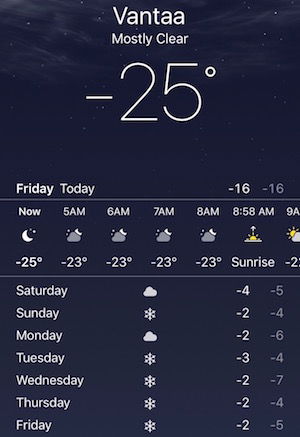Screenshot of a mobile weather application displaying the weather forecast for the city of Fanta. The screen has a sleek black background with white text for readability. At the top of the page, it reads "Fanta," indicating the city name. Below that, the current weather is described as "Mostly Clear" with a chilling temperature of -25 degrees. The day is identified as "Friday," with today's high expected to be -16 degrees.

The hourly forecast spans from the current time, which appears to be the middle of the night, through 9 a.m. It shows a noticeable temperature drop throughout the day. Further down, a brief weekly forecast illustrates the weather conditions from Saturday through Friday, highlighting anticipated snowfall on Sunday, and from Tuesday to Friday.